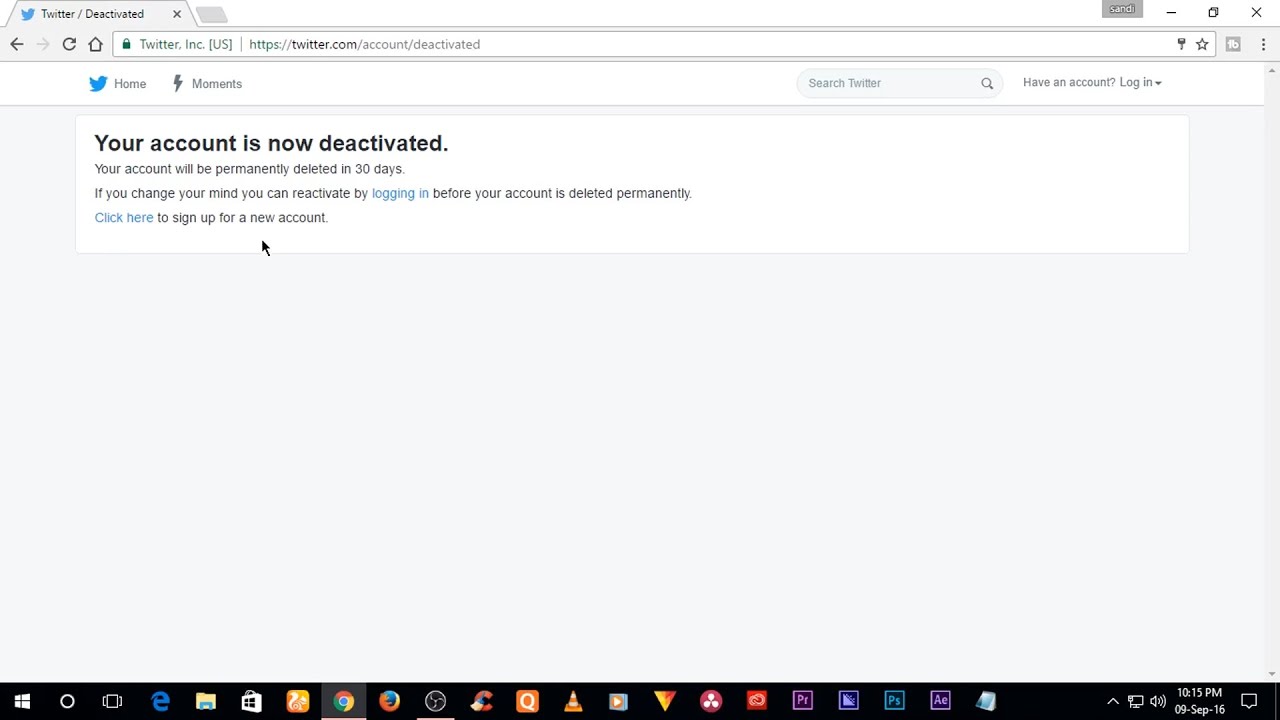The image depicts a web browser window displaying a deactivation confirmation page on Twitter. The top part shows an open browser tab, featuring the blue Twitter bird icon and the text "Black Twitter / Deactivated." To the left of the tab title, there is a dark grey left-pointing arrow, and to the right, a light grey right-pointing arrow, accompanied by a black circular arrow symbol for refreshing the page. 

Below the tab, within the white browser area, the URL bar displays "twitter.com" in green, followed by "/US", "https://", and "twitter.com/account/deactivated" in black and grey text.

Within the main content area, centered under another Twitter bird logo and navigation paths such as "Home" and "Moments," there is a prominent white box on a grey background. In bold black text, it states, "Your account is now deactivated. Your account will permanently be deleted in 30 days. If you change your mind, you can deactivate by logging in," with "logging in" rendered in blue as a clickable link. The text continues in black, explaining, "before your account is deleted permanently." A blue "click here" link follows, leading to the black text, "to sign up for a new account."

At the bottom of the screen, various browser and application icons are visible, including Chrome, Firefox, Settings, Internet Explorer, and Adobe Photoshop.